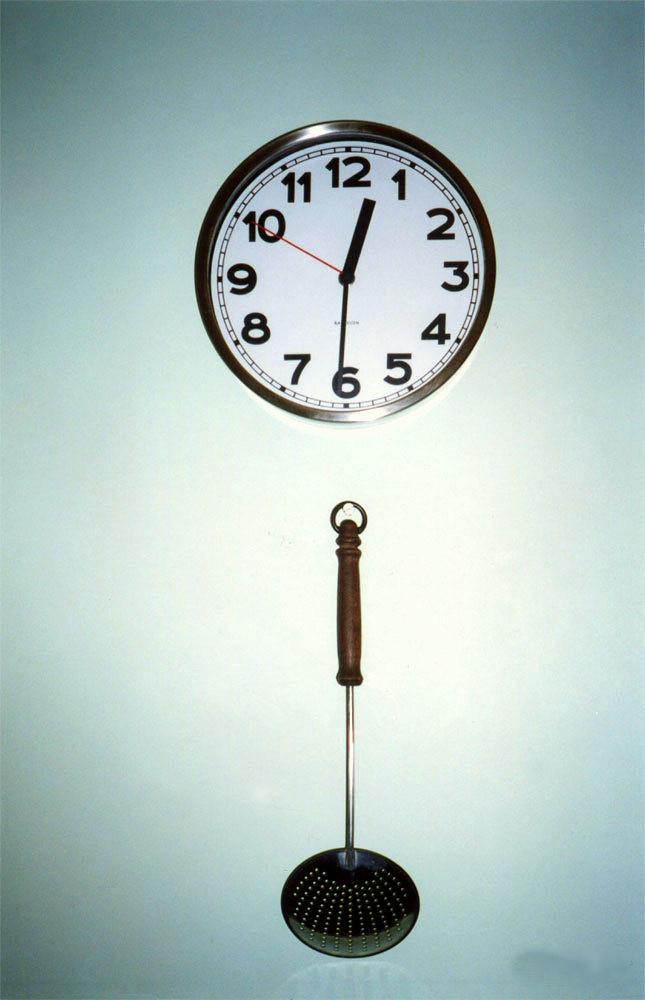In this photo, a round wall clock is hanging on a plain white wall, with its edges softly shadowed and the center slightly blurred due to a heavy flash. The clock features a dark edge, either black or brownish, while its face is white adorned with bold black numbers. The time displayed is 12:31, with a thick black hour hand, a thin black minute hand, and a striking red second hand pointing to the 10. Below the clock, a kitchen utensil is suspended by a nail, somewhat obscured by the flash. This utensil has a wooden handle that transitions into a metal shaft, terminating in a round, perforated end, suggesting it might be a strainer rather than a spatula. The utensil casts a shadow around its end, and the hook holding it, visible through the flash, appears to be a goldish hue.